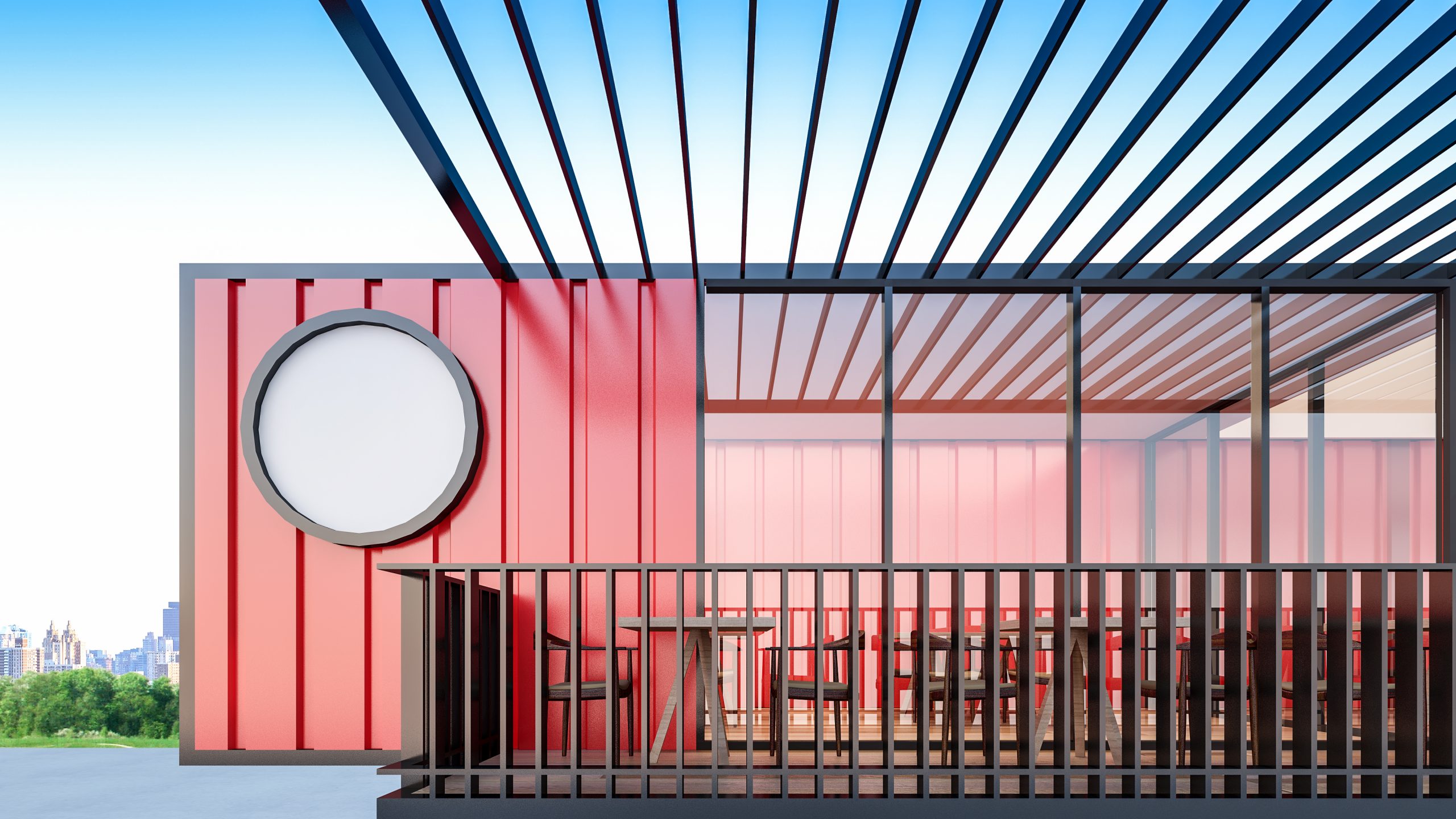This photograph captures a sunny day scene featuring a modern red building with a distinct architectural style. The building is divided into two sections: one half consists of large, tall windows that offer a glimpse into the building's interior, and the other half features a metallic-looking wall adorned with a giant white circle that could be either a window or an opaque decorative element. Adjacent to this wall is a small outdoor seating area, enclosed by a waist-high brown railing. The seating area contains a couple of tables and chairs, all made of brown wood, and is covered by a pergola with slats of dark brown wood running perpendicular to the seating area. In the background, beyond the building, one can see a clear blue sky, green trees, and the distant outline of a city skyline.